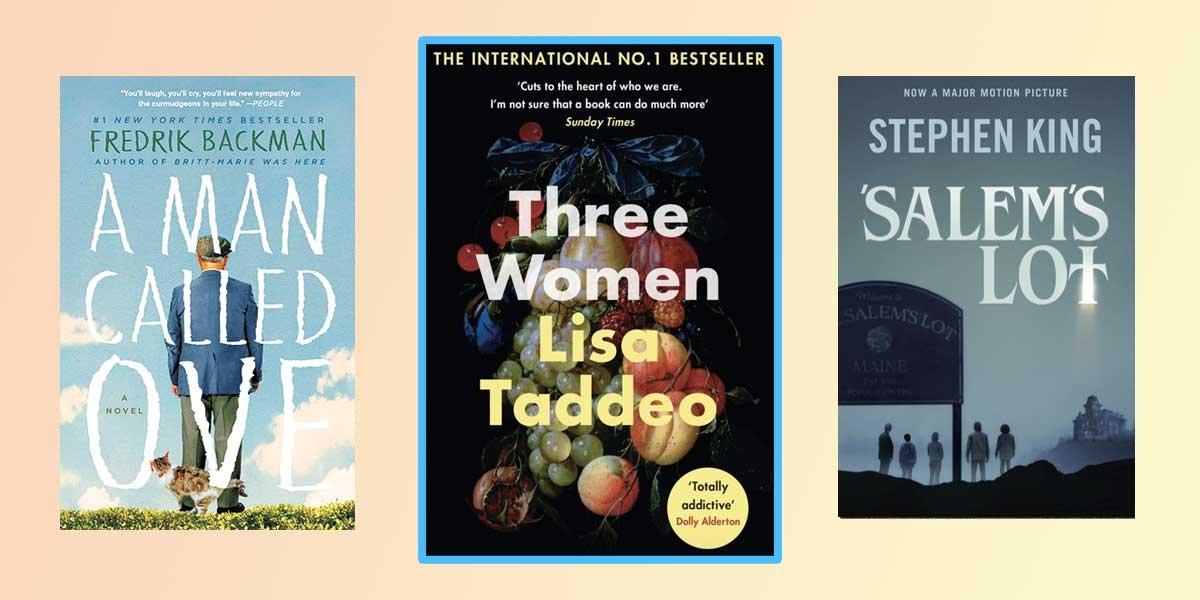The photo showcases three different books against a predominantly pink background. The first book on the left is "A Man Called Ove" by Fredrik Backman. Its cover features a man facing away from the viewer, standing on green grass under a blue sky with scattered clouds. At his feet is a cat. The middle book, prominently highlighted as an international number one bestseller, is "Three Women" by Lisa Taddeo. Its cover displays a dark background adorned with a vibrant assortment of fruit including peaches, grapes, blueberries, and plums. The third book on the right is "Salem's Lot" by Stephen King, which has a monochromatic, black-and-white cover and is now a major motion picture, suggesting a horror theme. The books are arranged neatly within a rectangular frame that transitions from a clear color to shades of peach and yellow, integrating seamlessly with the pink backdrop.